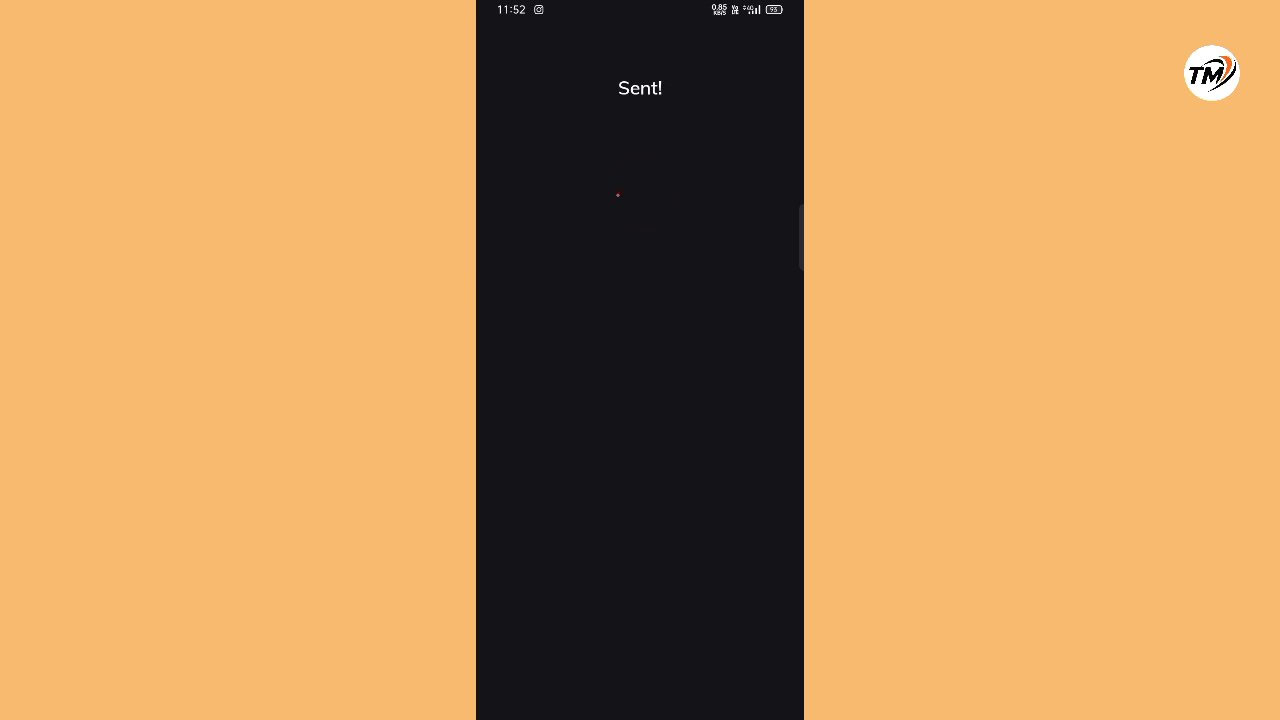The image depicts a black smartphone screen in portrait orientation, positioned at the center of a horizontal frame with a peach or light orange background. The black screen, resembling the dimensions of a smartphone screenshot, features small white text in the upper left corner indicating the time, "1152," followed by additional icons related to smartphone status like Wi-Fi or battery life in the upper right. Prominently, at the top of the black area, the white text "sent!" is displayed with an exclamation point. On the peach background's upper right corner, a white circular logo bearing the italicized black letters "TM" is visible, accompanied by curved arcs in orange and brown colors emanating from the circle. The composition lends a minimalist yet detailed representation reflective of photographic realism.